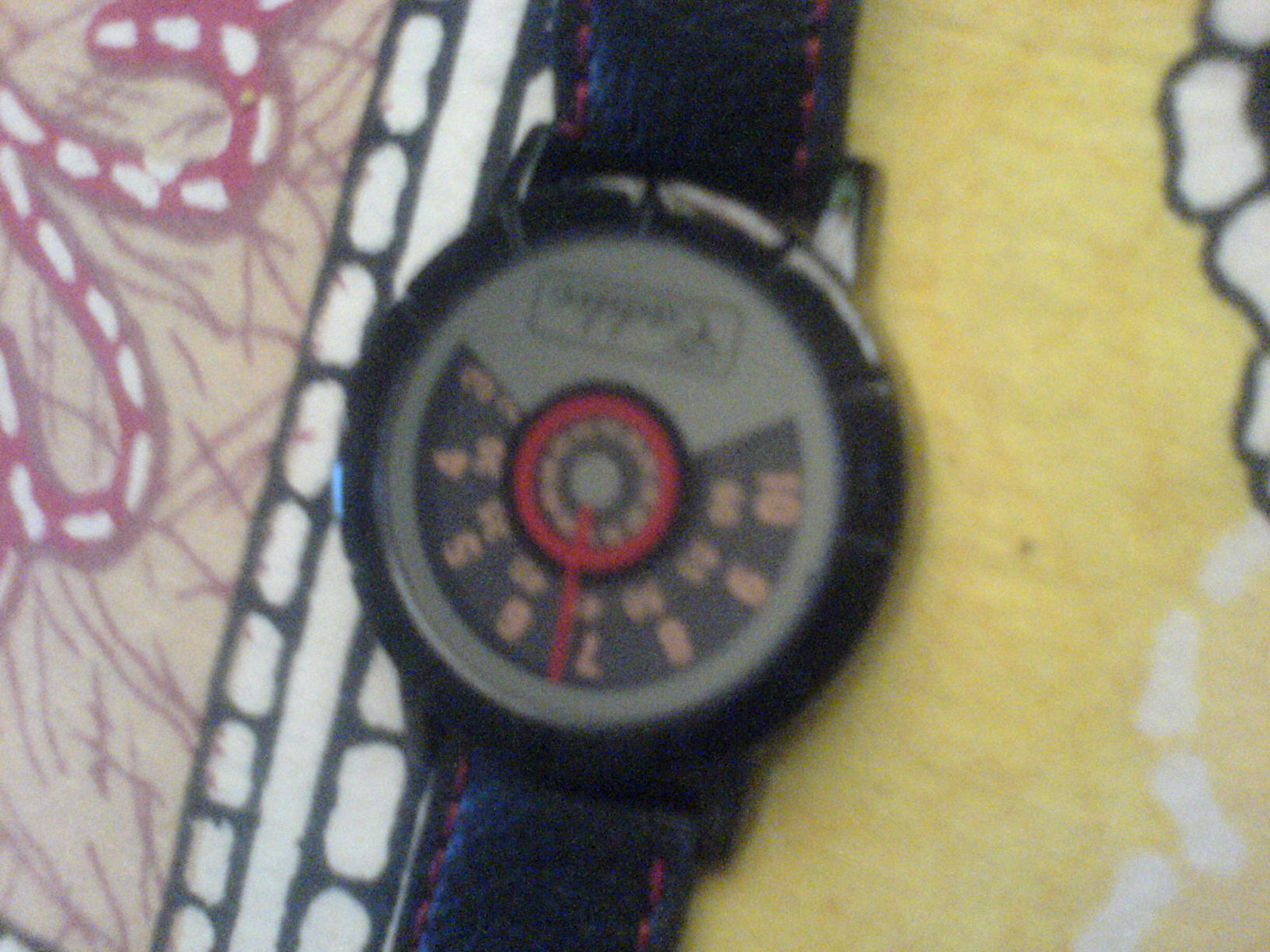This slightly out-of-focus photograph depicts an unorthodox wristwatch resting on a light brown or tan wooden surface. The watch, which appears to be turned upside down, features a black band. Its face is divided into distinctive sections: the outer black dial displays pinkish-yellow or orange-colored numbers ranging from 4 to 10, arranged in a semi-circle. The watch has a single red hand that rotates around a red center. Closer to the center, there are multiple circles, including a red inner circle and pink blotches that make it difficult to discern their exact nature. There is also some indistinguishable text within a box, likely indicating the model or manufacturer of the watch. Surrounding the watch on the left side is a diagram with red and white spots, possibly resembling candy canes and an old-timey tape pattern. On the right side, there is another white and black diagram that could be a drawing of a flower, while yellow shapes that resemble bones add to the textured background.